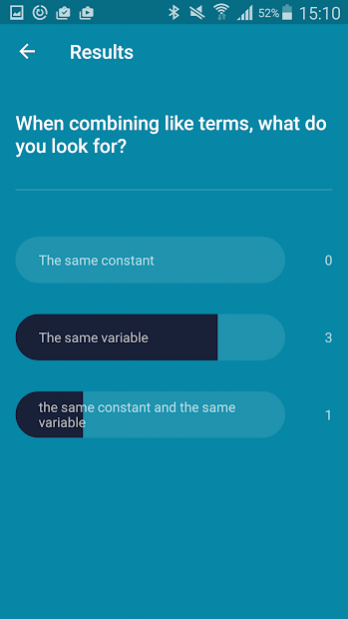A detailed view of a mobile phone screenshot displaying a results page within an app. At the top left corner, there are several icons: a photo icon, a refresh icon, a checkmark inside a briefcase, and a play button within a briefcase. The screen's top blue border also features various status icons: Bluetooth, sound turned off, full Wi-Fi bars, full data signal bars, and a battery life indicator at 52%. The time displayed is 15:10.

Beneath the border, the blue section contains white text and symbols, including a back arrow in the upper left corner. The main content area is titled “Results” and presents a question about combining like terms. There are three answer options listed: “the same constant with zero,” “the same variable with three,” and “the same constant and the same variable with one.”